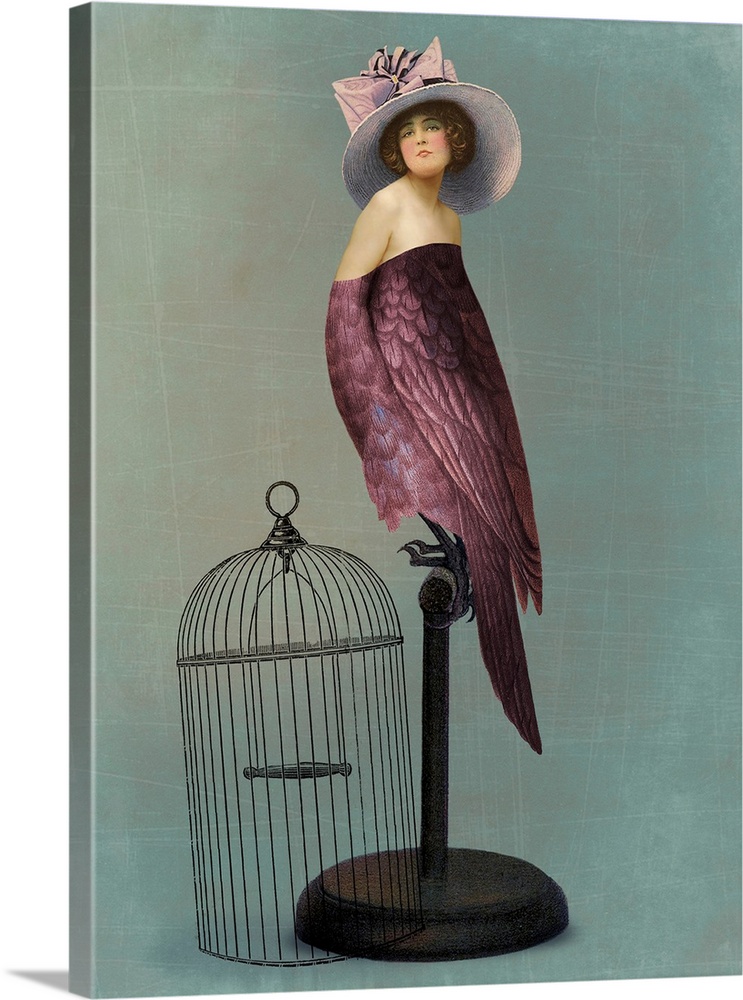The image features an abstract painting rendered on a canvas with a flat greenish-teal background adorned with various white scratches. Central to the composition is a fantastical figure perched on an antique bird stand with a circular black base and a vertical rod. This merged creature exhibits the lower body of a bird, detailed with purplish feathers, talons clutching the perch, and a bird's breast and tail. Transitioning to the upper half, the figure transforms into a woman reminiscent of the 1920s or 30s, characterized by her curly brown hair and heavily made-up pink cheeks. She wears a wide-brimmed hat accented with a purple bow. Adjacent to the perch lies a thin metal birdcage with a circular ring handle, suggesting she once resided within. The overall effect is a surreal blend of human and avian elements, playing with both time and form.